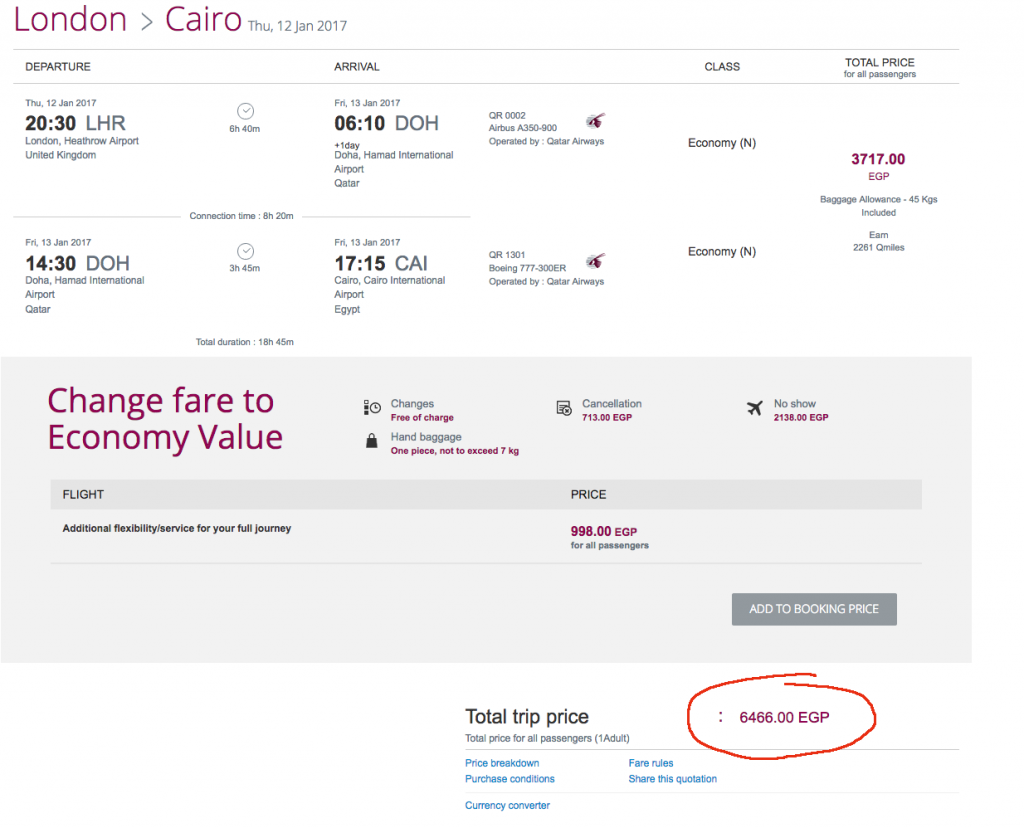This screenshot displays a detailed itinerary for an airline journey from London to Cairo. The flight is scheduled for Thursday, January 12, 2017. The departure time from London Heathrow (LHR) is 20:30, flight number LHR 610, with a connection time in Doha (DOH) of 14 hours and 30 minutes. The subsequent flight from Doha departs at 17:15 and arrives in Cairo (CAI). Both segments are in economy class. 

The ticket price for this itinerary is listed as 3,717 EGP. The baggage allowance for this trip is 45 kilograms. Additionally, passengers can earn 2,261 Qmiles. There are other fares available, such as changing to "Economy Value." The total trip price amounts to 6,466 EGP.